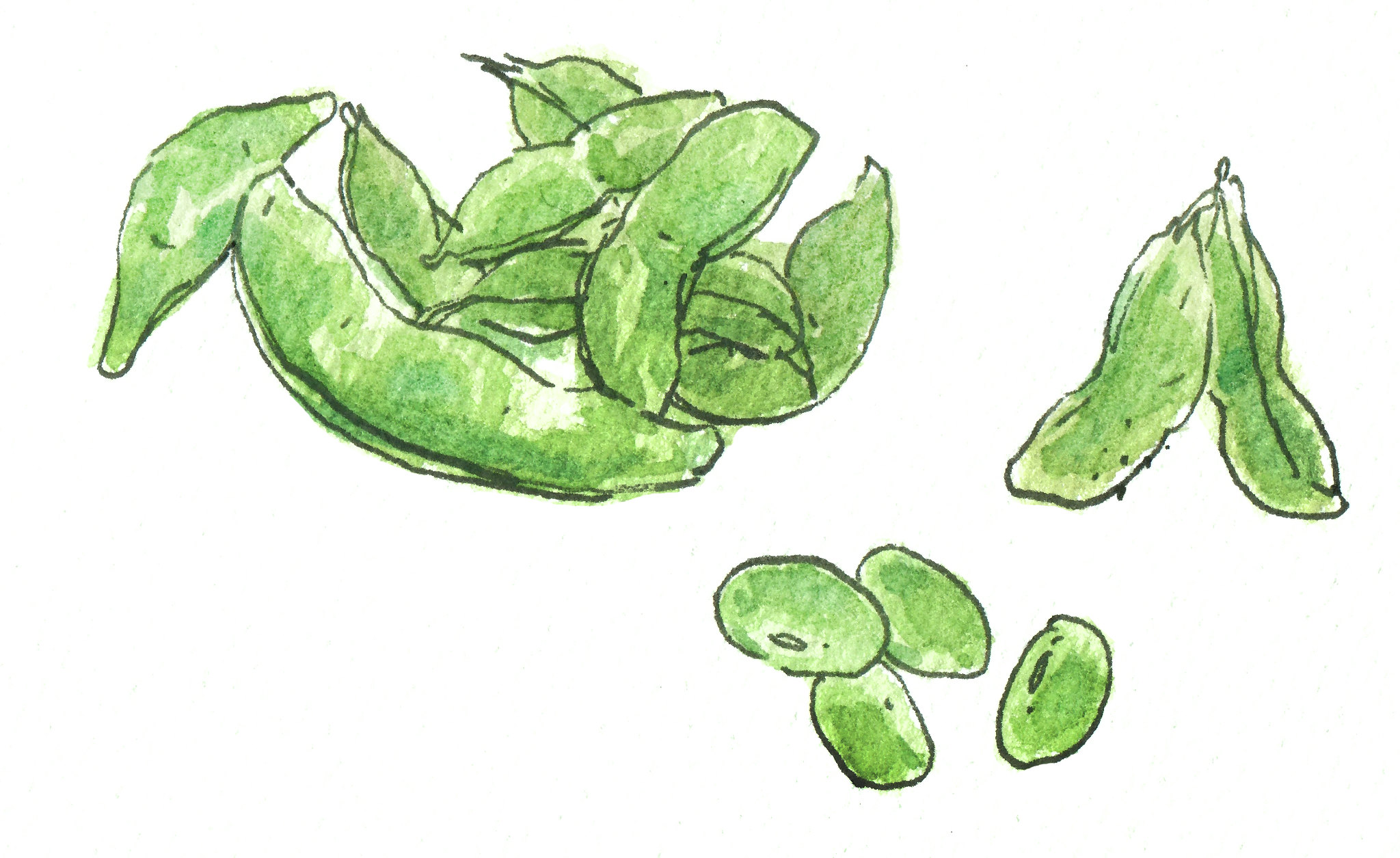This image depicts a detailed artistic drawing of green beans, primarily in green hues suggesting the use of watercolor and pencil, against an off-white background. The composition features a prominent cluster of approximately eight green beans in the top-left corner, stacked and interleaved at varying angles, some positioned diagonally and others laid flat. Two beans are seen propped against each other in the top-right corner, still connected by their stems. The bottom section of the image shows four individual beans that have been shelled. The artwork captures intricate details such as the indentations along the beans and subtle white highlights emphasizing their natural texture. The overall style is minimalistic, with fine black lines outlining the forms and a clear, untextured background, suggesting the medium could be a scanned or photographed watercolor piece.